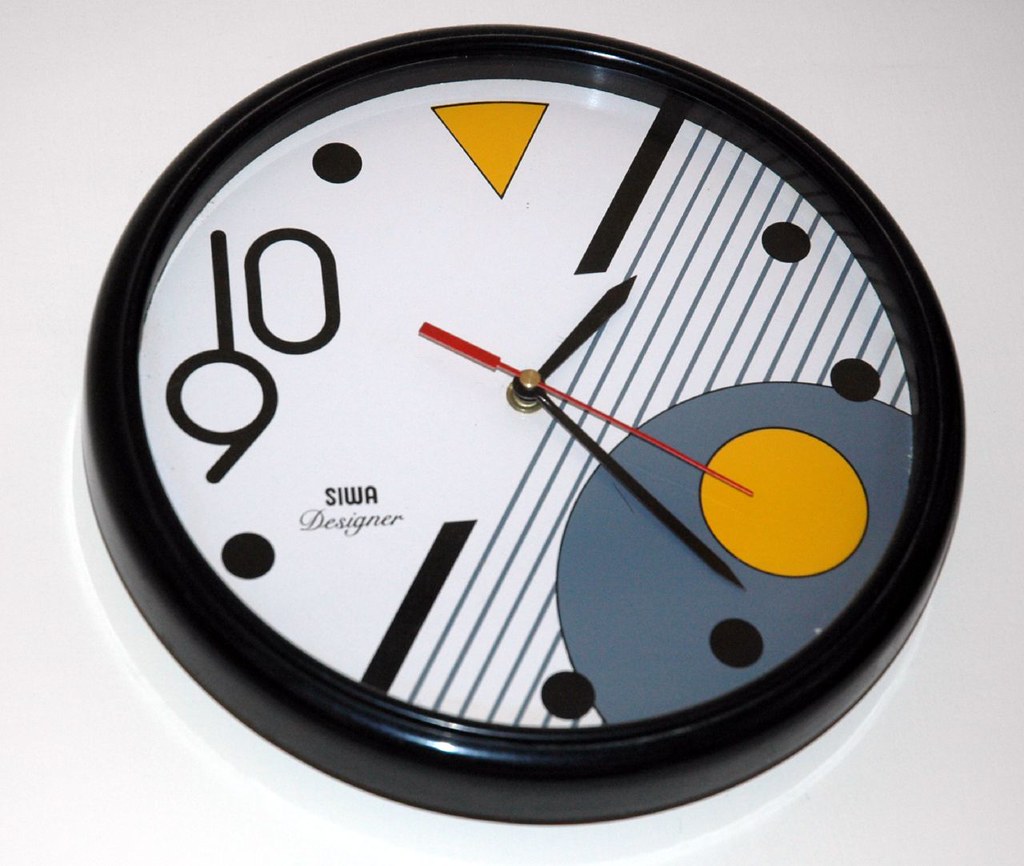This image features a uniquely designed clock hanging on a gray wall. The clock's outer edge is black, creating a bold frame for its eclectic face. The clock face is divided into two sections: the right half showcases gray stripes interspersed with dots that mark the hours, while the left half has a white background. Distinctive hour markers include a large yellow dot, several black dots, and an equilateral yellow triangle pointing downward that denotes the 12 o'clock position. Unlike traditional clocks, the only numerals present are "10" and "9," located on the left-hand side. There are also two dots—one below the "9" and one above the "10"—which presumably indicate the 11 o'clock position. The clock hands are black, except for the second hand, which is red, adding a subtle pop of color. The words "SIWA Designer" are inscribed on the clock face, emphasizing its modern and artistic design.